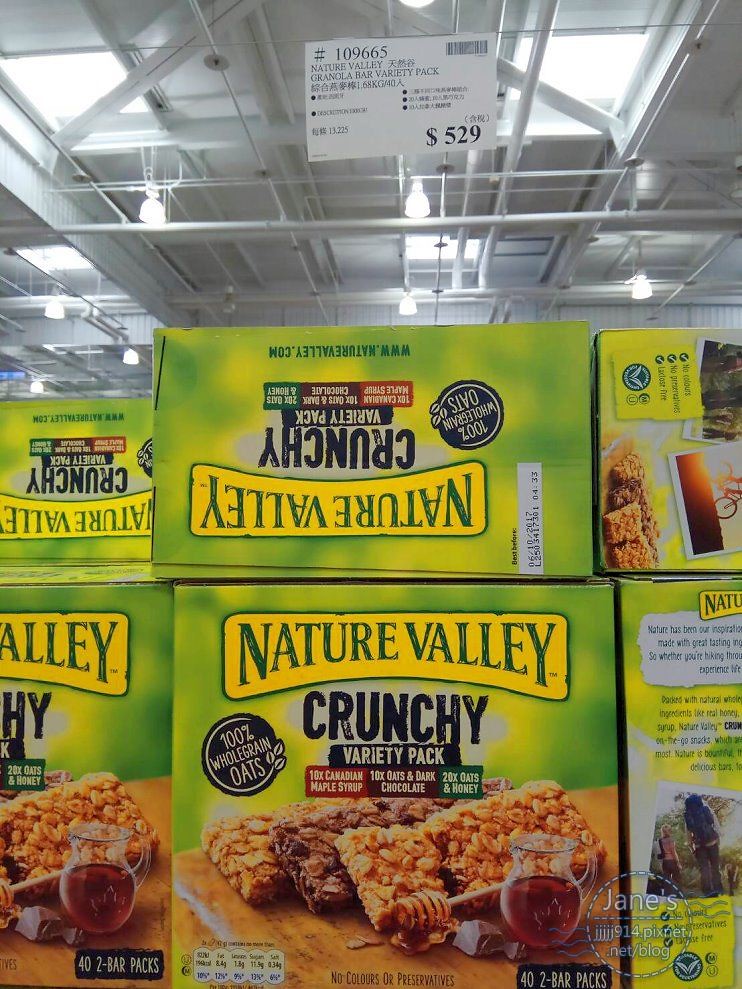The image captures the interior of a large warehouse-like store, reminiscent of Costco. At the top portion of the image, the ceiling rafters and beams stretch out, with skylights positioned to the left and right, casting light into the space. Dominating the scene is a large white poster hanging from the ceiling, though its text is unreadable. Centrally featured in the foreground are boxes of Nature Valley Crunchy Granola Bars, specifically the variety pack which includes images of the granola bars and three different flavors—original, chocolate, and an indistinct third type. The box design is green, highlighting the product in an eye-catching manner indicative of bulk buying. Two boxes are prominently stacked in the center, surrounded by partially visible boxes cropped by the image's edges. Notably, a faint white circle containing the word "Janes" is located in the bottom right corner. Above the granola bar display, an informational sign reads "$529," presumably unrelated to the granola bars themselves, suggesting the price is for an item in a different location. The overall setting, visual elements, and product details create the impression of a spacious, well-lit store environment.